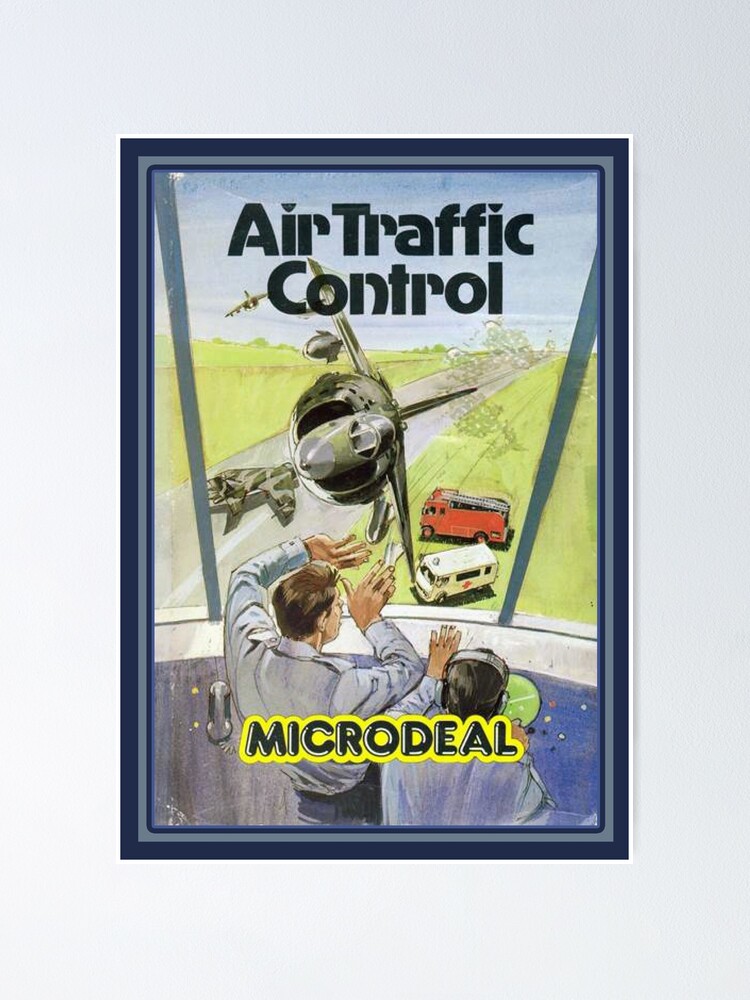This image captures a vintage poster, potentially from the 80s or 90s, depicting an intense scene at an air traffic control center. Two employees, dressed in blue shirts with panicked expressions, have their hands raised in alarm as a large, greenish-gray camouflaged fighter jet veers dangerously close to the tower window. The title "Air Traffic Control" is prominently displayed at the top in heavy black font. Below the console area, which features radar equipment and an old phone handset, the words "Micro Deal" stand out in bold, black 3D letters with a yellow outline. Through the elevated tower window, emergency vehicles, including a short fire truck and a white ambulance with a red cross, are visible on the ground. The runway stretches from the foreground to the upper right, where a military plane appears to be taking off. Additionally, another jet is seen airborne in the distant sky. The overall scene combines elements of urgency and chaos, set against a white or slightly gray-toned drywall backdrop.